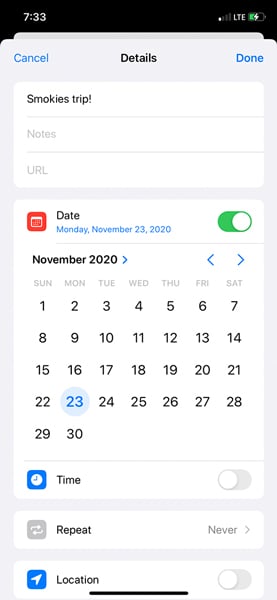The image showcases a phone screenshot with intricate details. At the top of the screen, a black status bar is visible, featuring grey text. On the left side of the bar, the time "7:33" is displayed. To the right, a single cell phone signal bar, the notation "LTE," and a green battery icon indicating charging are shown.

Below the status bar, the primary part of the screen appears in grey. At the top left, the word "Cancel" is in blue text, with "Details" in black text at the center and "Done" in blue on the right. The title "Smokey's Trip!" is prominently displayed in white text, followed by a section labeled "Notes" in black text. Presently, no URL is specified in the URL field.

A calendar interface is displayed next, characterized by a small red box with a black calendar icon in the upper left corner. The text "Date" in red is adjacent to it. The date "Monday, November 3rd, 2020" is highlighted in blue.

Beneath this are navigational elements for the month of November 2020, featuring left and right arrows in blue, accompanying the text. The days of the week (Sun, Mon, Tues, Wednes, Thurs, Fri, Sat) are shown in grey, with the calendar days in black text. Notably, "Monday, November 23rd" is highlighted in grey with blue text.

Further down, the section labeled "Time" is in black, accompanied by a blue clock icon. The "Repeat" setting is turned off, and the "Location" setting is enabled, indicated by a blue GPS icon. At the very bottom center of the page, a small black bar is visible.

This detailed screenshot captures various information such as time, date, calendar settings, and other relevant details associated with "Smokey's Trip!" event.